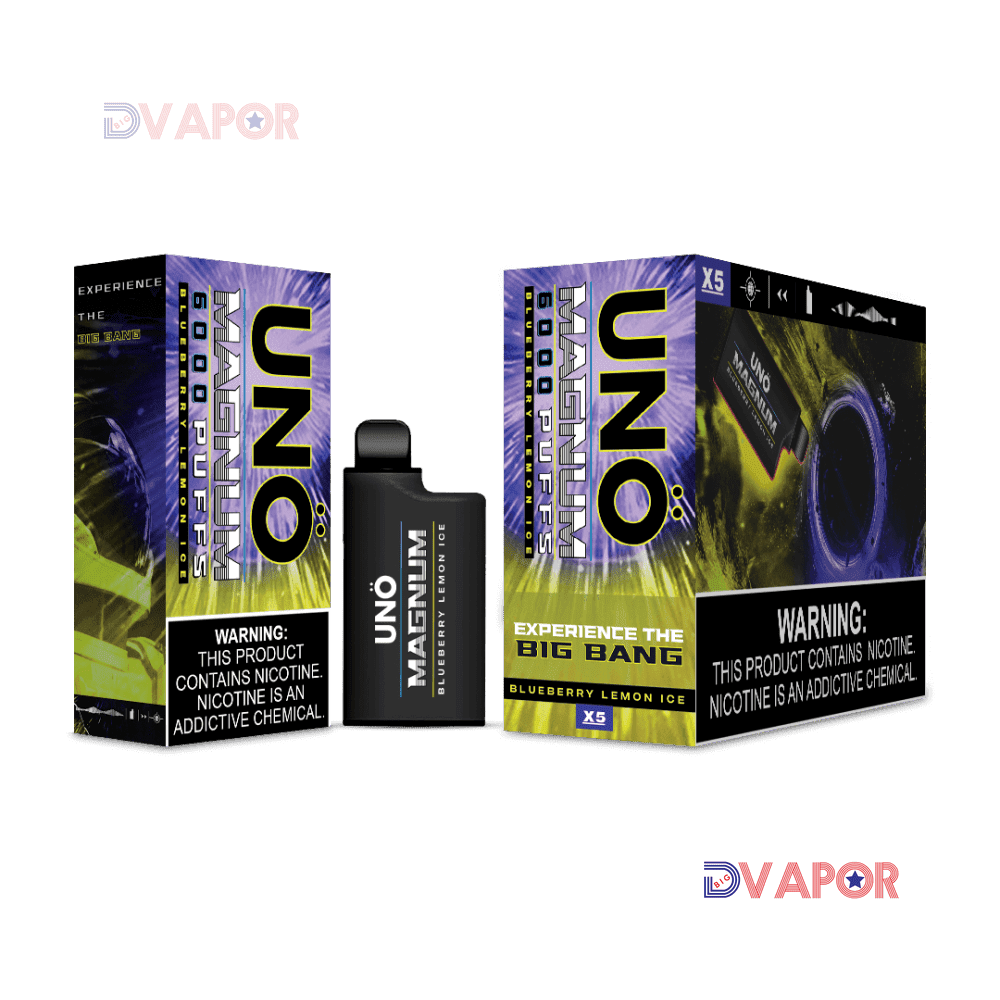The image displays a detailed ad for a product called UNO Magnum by D Vapor, set against a white background. Prominently, it features two boxes and a canister-like vape device situated in the center. The vape device, black and resembling a gun magazine clip, showcases the label "UNO Magnum Blueberry Lemon Ice" in white font. The boxes, both featuring a vibrant design with a purple burst at the top and yellowish bottom, contain similar labels. 

The box on the left is taller and narrower, while the box on the right is shorter but deeper. Each box includes bold white warning text at the bottom, stating, "WARNING: This product contains nicotine. Nicotine is an addictive chemical." These warnings are underscored for emphasis. Additionally, the tagline "Experience the Big Bang" is partially visible on the side of one of the boxes. 

The UNO and Magnum words stand out, designed to evoke an explosive visual theme. Also noteworthy, a watermark reading "DVAPOR" (with "D" in blue and "VAPOR" in red, accompanied by a blue star on the 'O') is placed at the top left and lower right corners. The overall design hints at a robust and dynamic vaping experience, with 6,000 puffs of Blueberry Lemon Ice flavor, as indicated on the packaging.